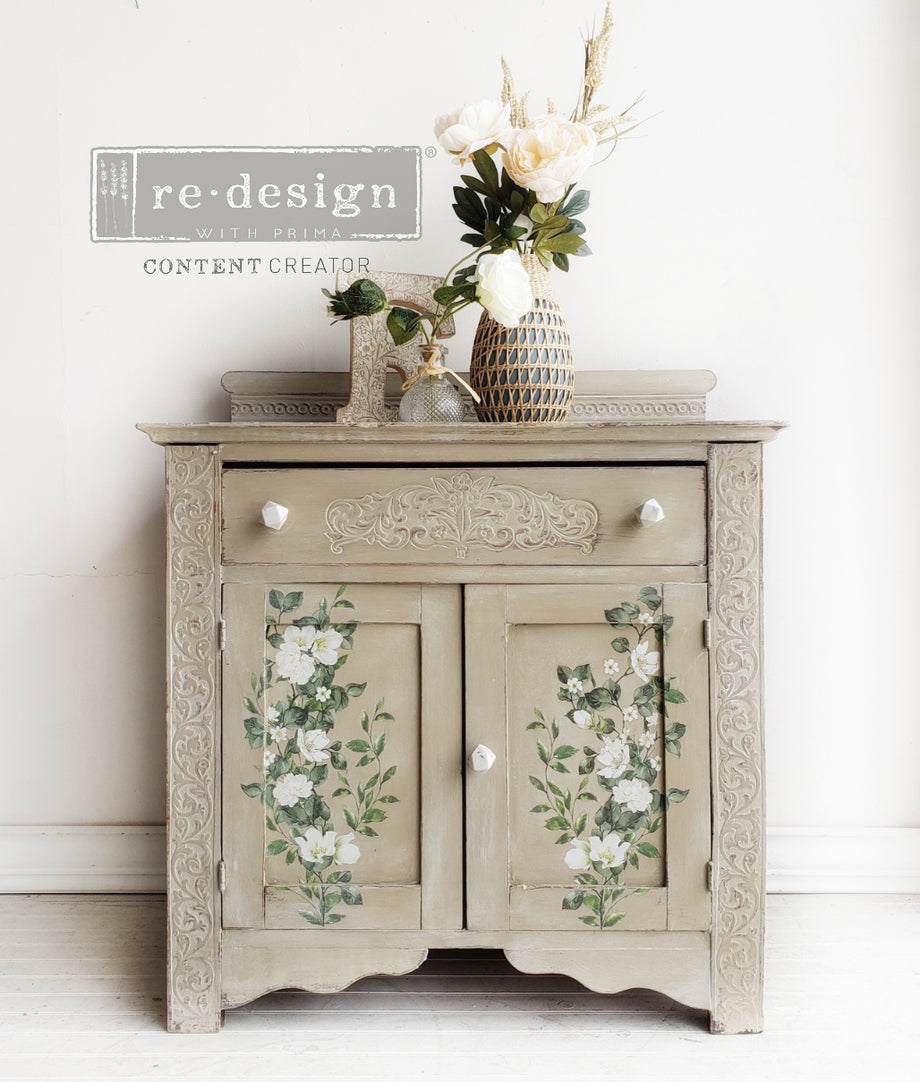This detailed advertisement image showcases a beautifully redesigned cabinet set against a stark white wall, creating a striking visual contrast. The cabinet itself is primarily gray with an elegant scroll pattern adorning the sides and borders. The front features a horizontal drawer with two white knobs and vertical cabinet doors that boast intricate designs of white flowers with green leaves and vines. Atop the cabinet, there's a sophisticated arrangement including a large, textured vase brimming with white peonies, a clear small vase with leafy sprigs, and a decorative, carved letter "F". The advertisement prominently features the label "Redesign with Prima" and "Content Creator" in gray and white lettering on the wall, subtly marking the branding. The floor beneath the cabinet has a patterned design, complementing the vintage aesthetic of the piece.